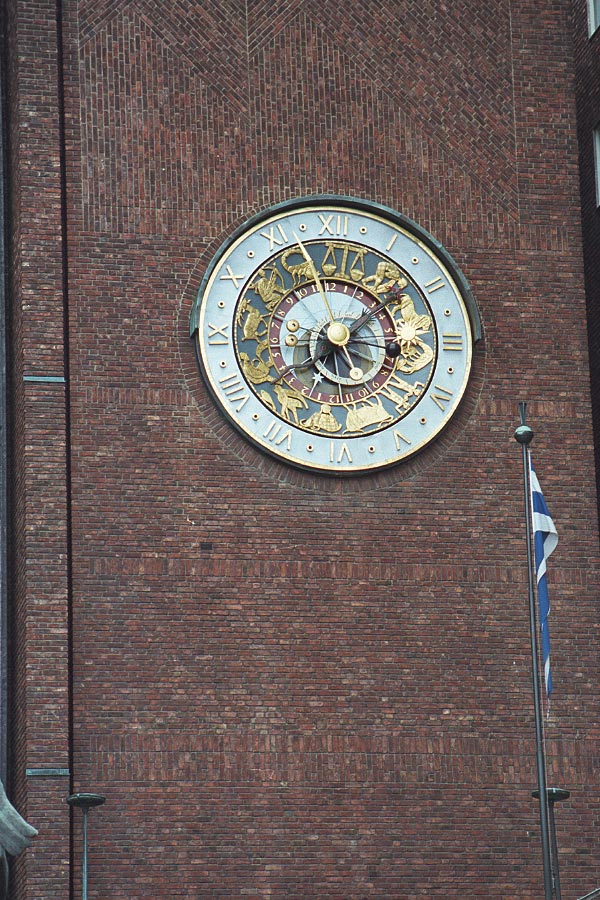An intricate image capturing the astronomical clock on Oslo City Hall. This imposing timepiece stands against the rustic backdrop of a brick façade. The clock itself is a splendid juxtaposition of colors, featuring a prominent white face adorned with blue and gold accents. Roman numerals mark the hours on the clock, while delicate gold and black hands point to the current time, which reads precisely 5:56. Surrounding the numbers are an array of detailed zodiac symbols, including the scales of justice, a scorpion, an archer, and an ox, among others. A proud Norwegian flag flutters gracefully in the foreground, adding to the scene's patriotic charm. The overall composition beautifully marries historical artistry with national pride.